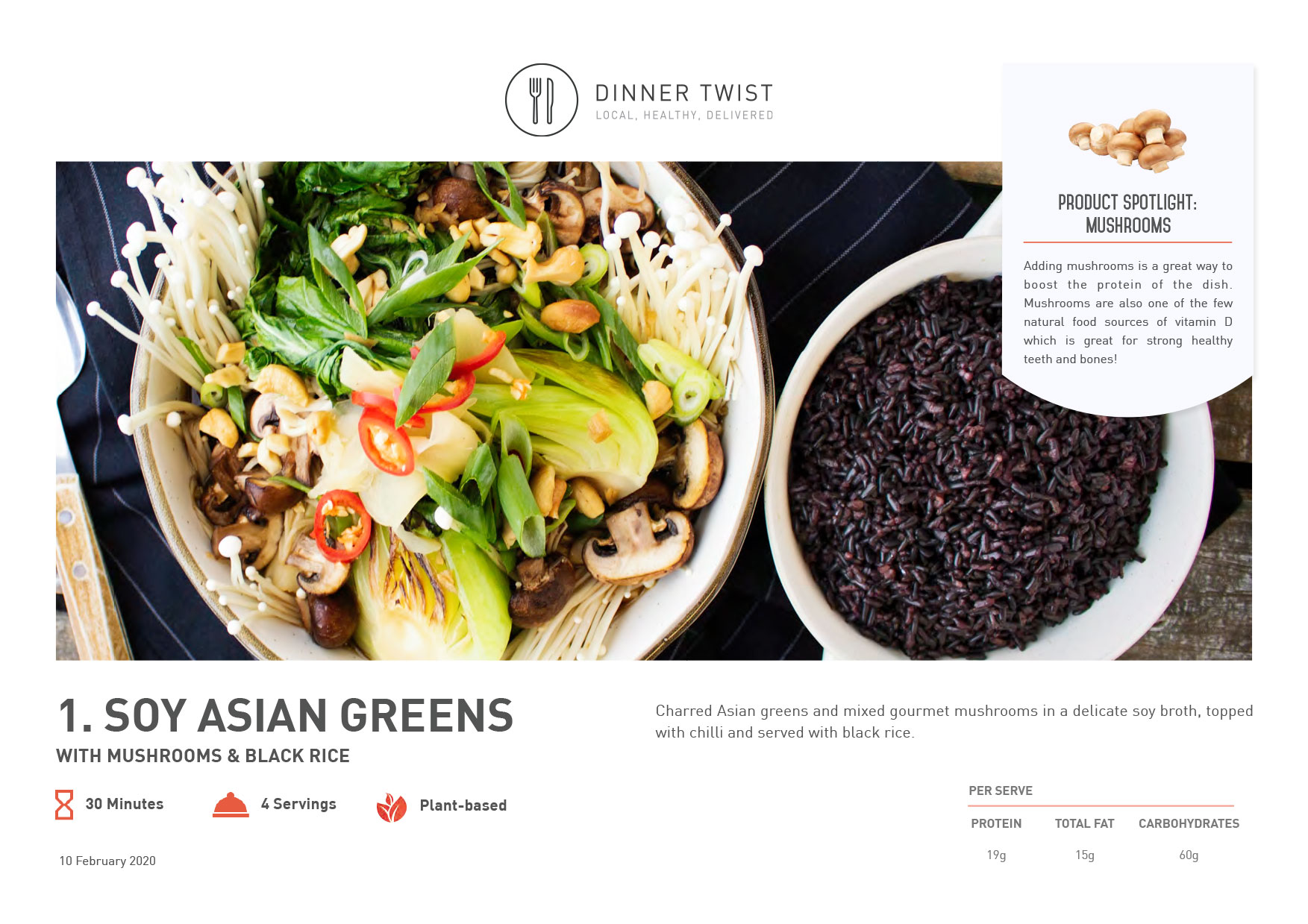This promotional image for Dinner Twist prominently features the tagline "Local, Healthy, Delivered." On the left side of the image is a vibrant bowl filled with an assortment of vegetables, nuts, and mushrooms. On the right, there's another bowl containing what appears to be dark-colored rice or beans. The right side also includes a "Product Spotlight" section focusing on mushrooms, highlighted as a great way to boost protein in a dish. It mentions that mushrooms are one of the few natural food sources of vitamin D, beneficial for maintaining strong, healthy teeth and bones.

Below this, it details the featured dish: "Soy Asian Greens with Mushrooms and Black Rice." The description reads: "Charred Asian greens and mixed gourmet mushrooms in a delicate soy broth, topped with chili and served with black rice." Icons indicate that the preparation time is 30 minutes, the dish yields four servings, and it is plant-based. The date "10 February, 2020" is noted at the lower section. Nutritional information per serving is listed as 19 grams of protein, 15 grams of total fat, and 60 grams of carbohydrates.